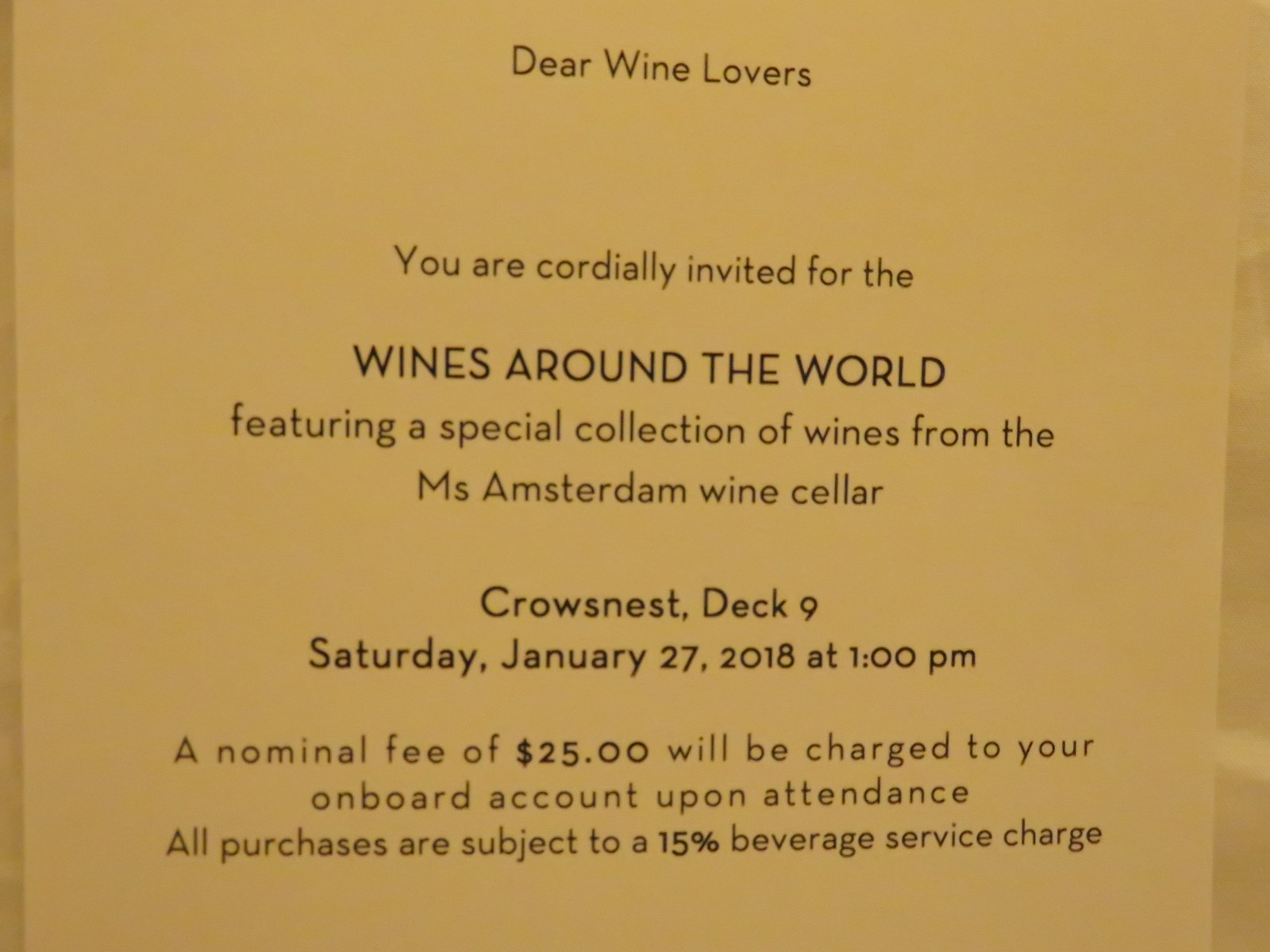This image depicts a yellow-tinted invitation card with a gold border, announcing an exclusive event titled "Wines Around the World." The text is primarily in black font and reads: "Dear Wine Lovers, You are cordially invited for the Wines Around the World, featuring a special collection of wines from the Ms. Amsterdam Wine Cellar. Crows Nest, Deck 9, Saturday, January 27th, 2018 at 1 PM." Notably, the event name, location, date, and costs are bolded for emphasis. The invitation also specifies that a nominal fee of $25 will be charged to attendees' onboard accounts upon attendance, and all purchases are subject to a 15% beverage service charge. Fine print includes a call to action for more information via the website, www.nsw.gov.au. This detailed text suggests the event is for cruise ship passengers, inviting them to partake in a curated wine tasting experience.